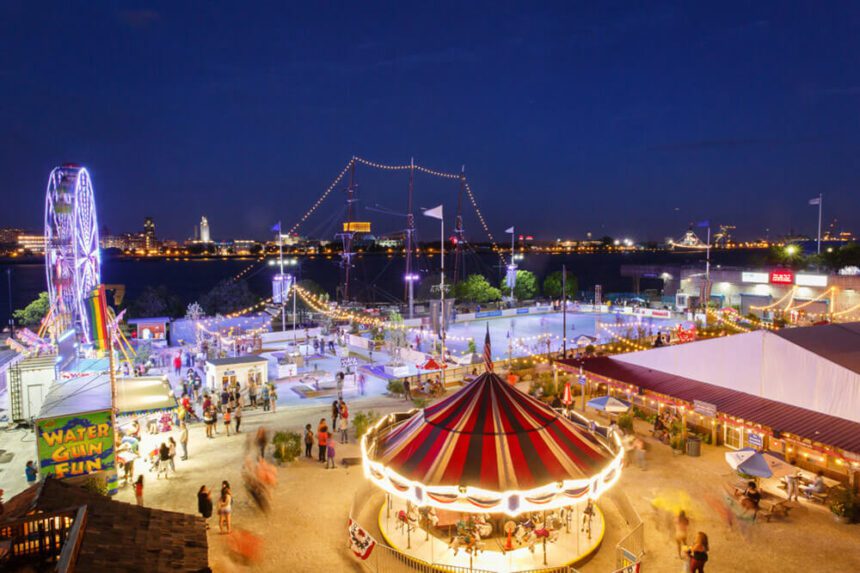This image presents an aerial view of a bustling carnival set against a backdrop of a deep blue twilight sky. Far in the distance, a cityscape adorned with twinkling lights stretches across the horizon. The carnival itself is situated near a large body of water, possibly suggesting a coastal location. 

In the foreground, at the center, a grand carousel draws attention with its vibrant red, white, and blue striped canopy, featuring horses and children riding them. Surrounding the carousel, clusters of people can be seen milling about, enjoying the lively atmosphere. 

To the right of the carousel, a brightly lit Ferris wheel adds to the festive ambiance. Nearby, an ice skating rink is enclosed by a white and blue board, its smooth surface reflecting the glow of the surrounding lights. 

On the left side of the image, a low building bears the sign "Water Gun Fun," indicating a game where people are likely engaged in shooting water guns. Adjacent to this, a building with a brown roof provides a sense of structure and perhaps houses refreshments or additional activities.

Scattered throughout the carnival are tables shaded by blue and white umbrellas, offering spots for visitors to rest and take in the sights. On the far right, a white building with a red roof stands, possibly a refreshment stand, adding to the array of attractions in this vibrant, evening scene.